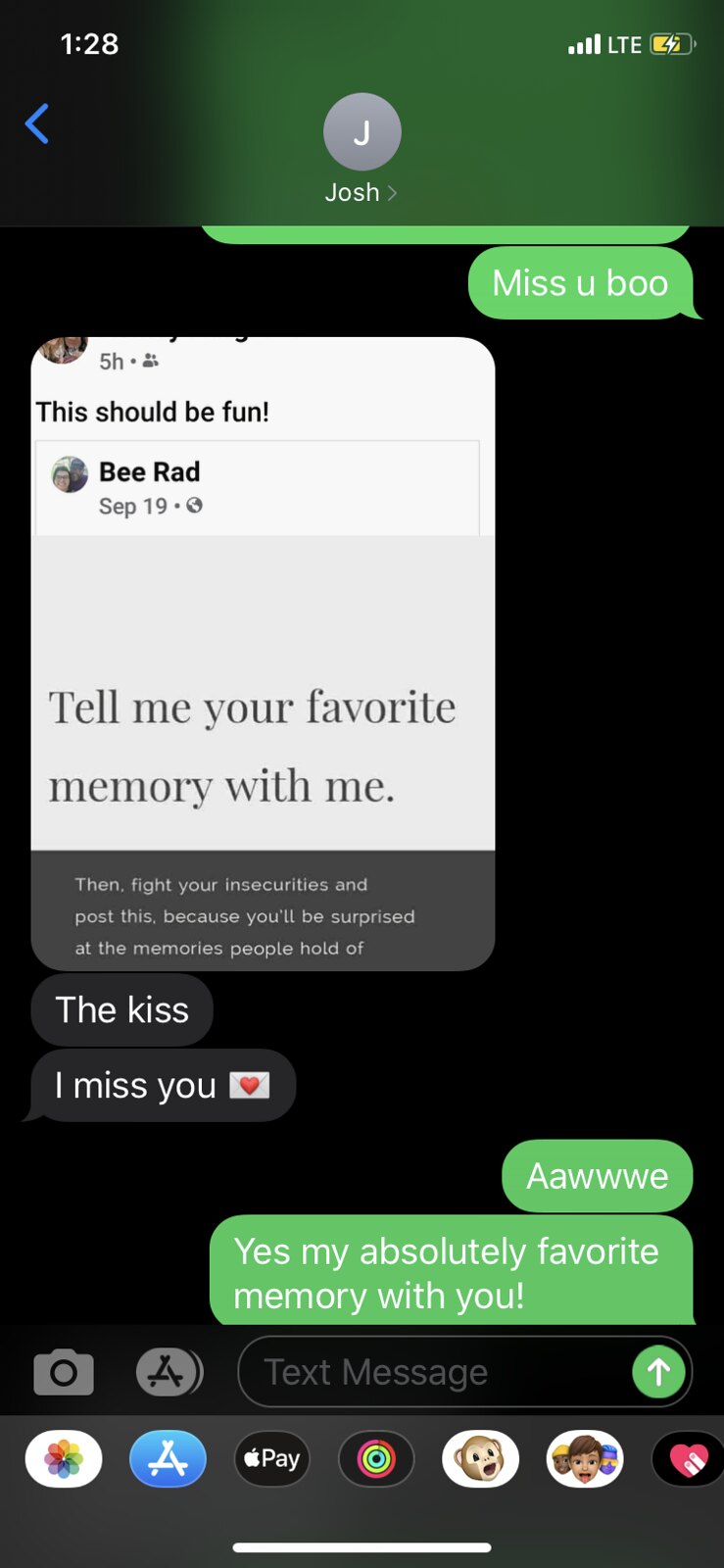The image is a screenshot taken from a smartphone, displaying a text message conversation between two people. The top of the screen shows the time as 1:28, with the signal strength indicating LTE mode and the battery about halfway charged. The contact name is Josh, represented by a silver circle with a white "J" in the top left. The conversation starts with a message in blue text saying "Miss You Boo." The reply in green text reads, "This should be fun, tell me your favorite memory with me," followed by, "The kiss, I miss you," accompanied by an envelope emoji with a heart. The final response, also in green text, states, "Aww, yes, my absolutely favorite memory with you." Below the conversation, the interface includes icons for apps and features, such as a camera, text input field, a green arrow for sending messages, and other icons like a heart, person, and emoji options on a black background.